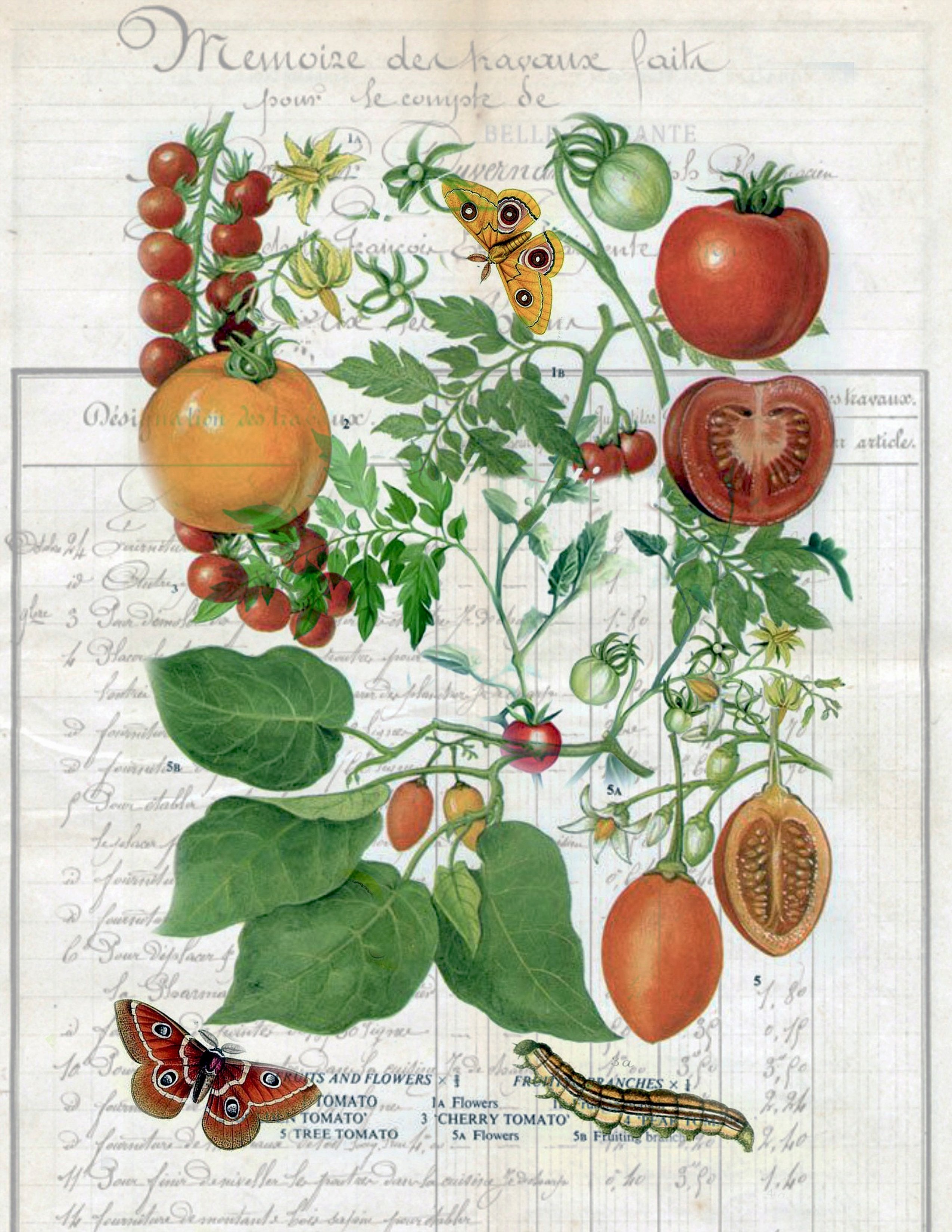This image features a detailed botanical guide to various tomato plants, set against an aged, grayish-white background that resembles a tally or account book filled with handwritten text in a foreign language. It includes beautiful illustrations of numerous types of tomatoes: red and orange round tomatoes, clusters of cherry tomatoes, Campari tomatoes, and plum-shaped tomatoes in various colors. Alongside the plants, the image depicts small green tomatoes on vines, assorted tomato leaves, and pests such as worms and caterpillars known to eat the tomatoes or their leaves. Prominently, there is also an orange moth or butterfly, possibly responsible for laying the eggs that hatch into these tomato-eating worms. The overall composition is a rich, informative visual on the diverse world of tomatoes and their pests.